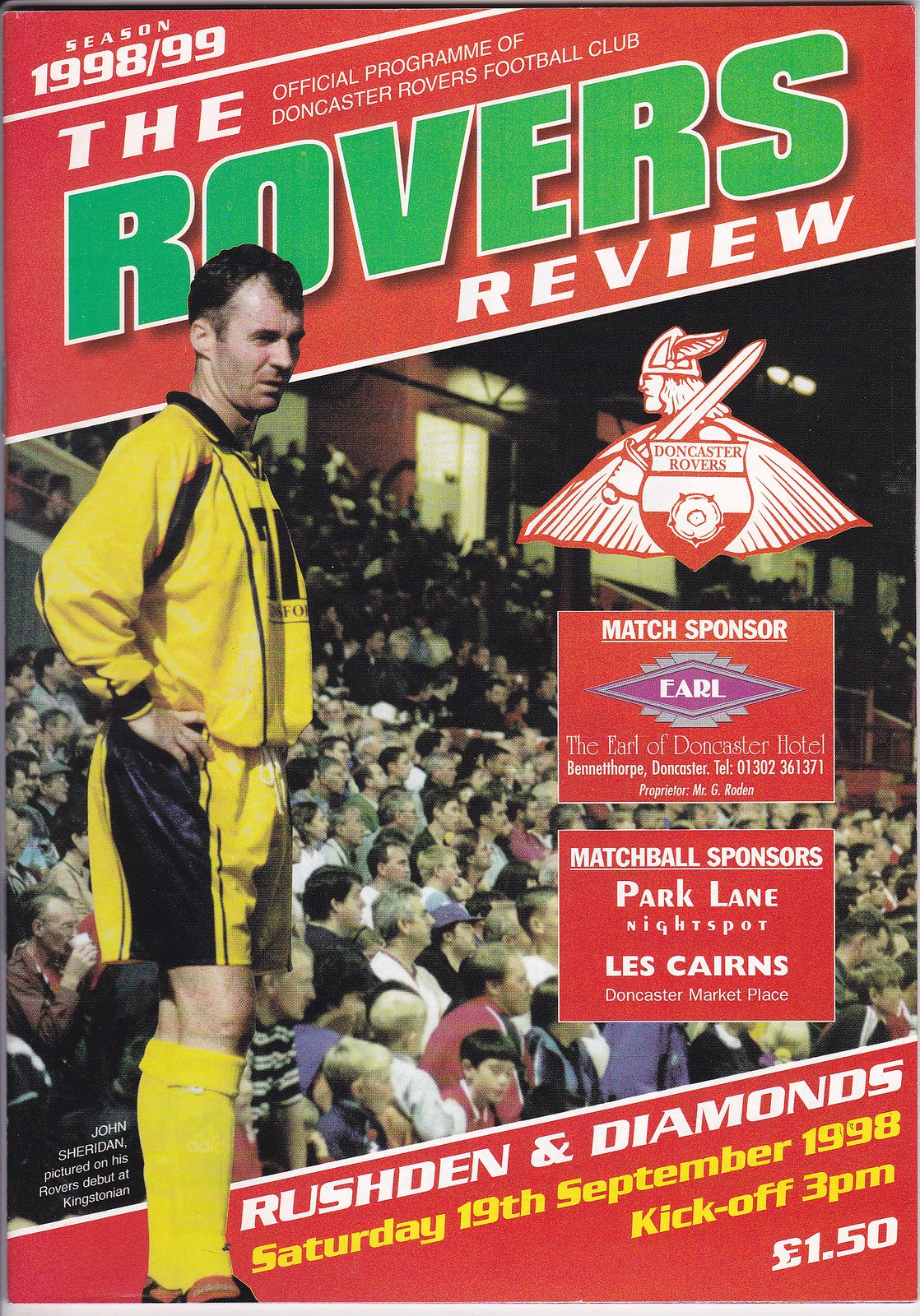The image is the front cover of a vertically oriented, red-background program for a sports game, specifically for Doncaster Rovers Football Club's 1998-99 season. In the top left corner, it states in white text, "Season 1998-99." Below that, in large green letters on a red banner, it reads "Rovers Review," followed by "The Official Program of Doncaster Rovers Football Club" also in white text. Dominating the left side of the cover is a full-length image of a man named John Sheridan, pictured in his Rovers debut at Kingstonian. He is wearing a yellow soccer jersey with black accents, including black numbers on the front, black and yellow shorts with a black stripe down the side, and yellow socks. Overlaying a crowd scene in the background, the crowd shot reveals fans in the bleachers watching a soccer match. To the right side of the cover, a logo of a Viking with a sword over his shoulder and a cape represents the Doncaster Rovers. Below this, there are details about the match sponsors: "Match Sponsors Earl, the Earl of Doncaster Hotel," and "Match Ball Sponsors Park Lane, Night Spot, Les Karnes, Doncaster Marketplace." In the lower right corner, there's a red banner that mentions "Rushden and Diamonds, Saturday, 19th September 1998, kickoff 3 o'clock p.m." The program is priced at £1.50.